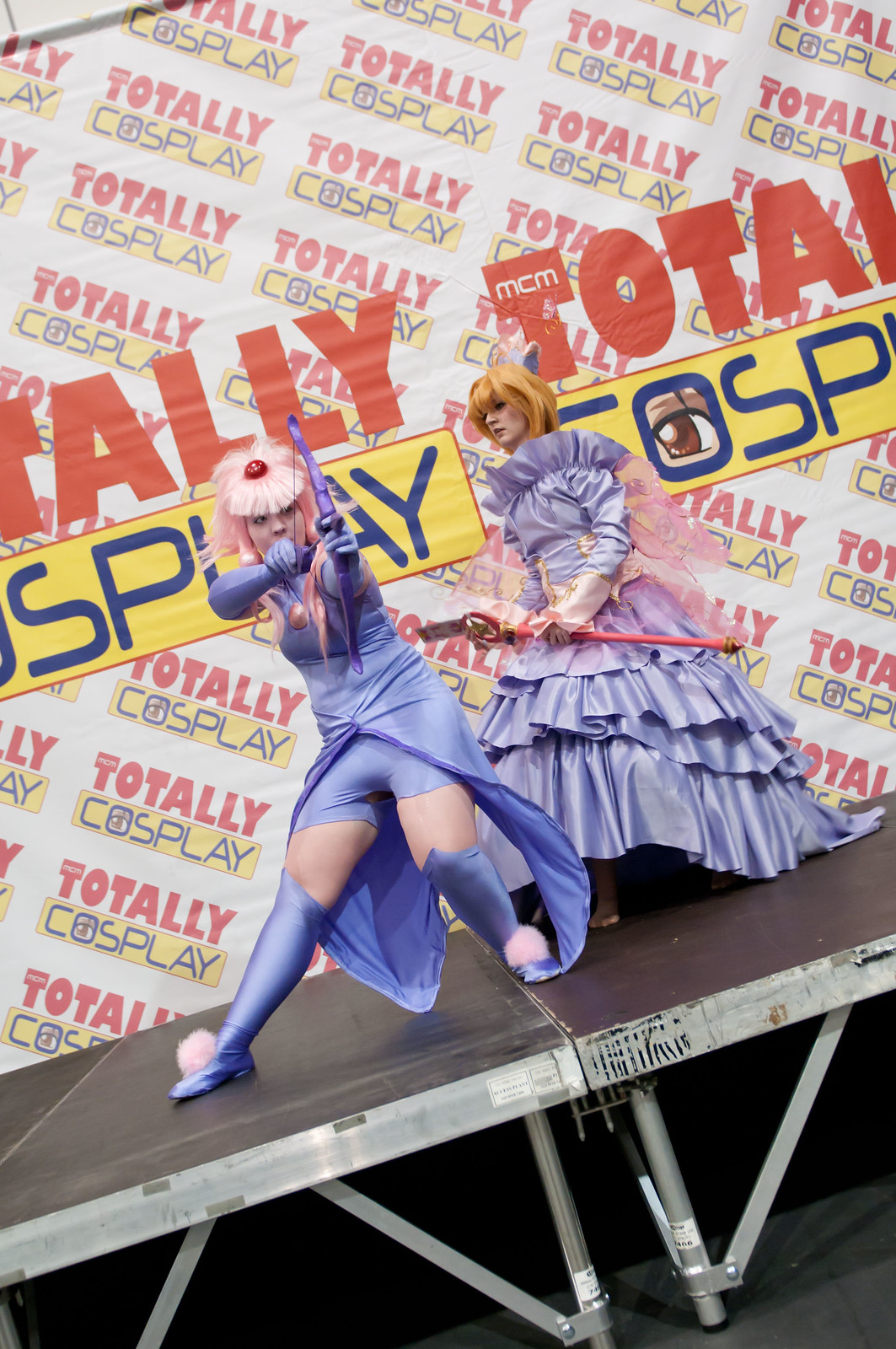The image depicts two individuals in elaborate costumes engaging in a lively performance on a stage. Both are dressed in vibrant blue-themed cosplay outfits, with one person donning a reddish-orange wig and the other sporting a pink wig. The stage, which has a brown top and a silver base, tilts slightly to the left in the photograph. Behind them hangs a large, colorful sign in white, red, yellow, and blue, declaring "Totally Cosplay." The person on the left wears knee-length blue satin boots with pink cotton balls on top, tight shorts, and a cape, while holding an unknown object. The person on the right is adorned in an intricate, layered blue silk dress, possibly holding a folded parasol, giving an impression of high glamour and whimsy.